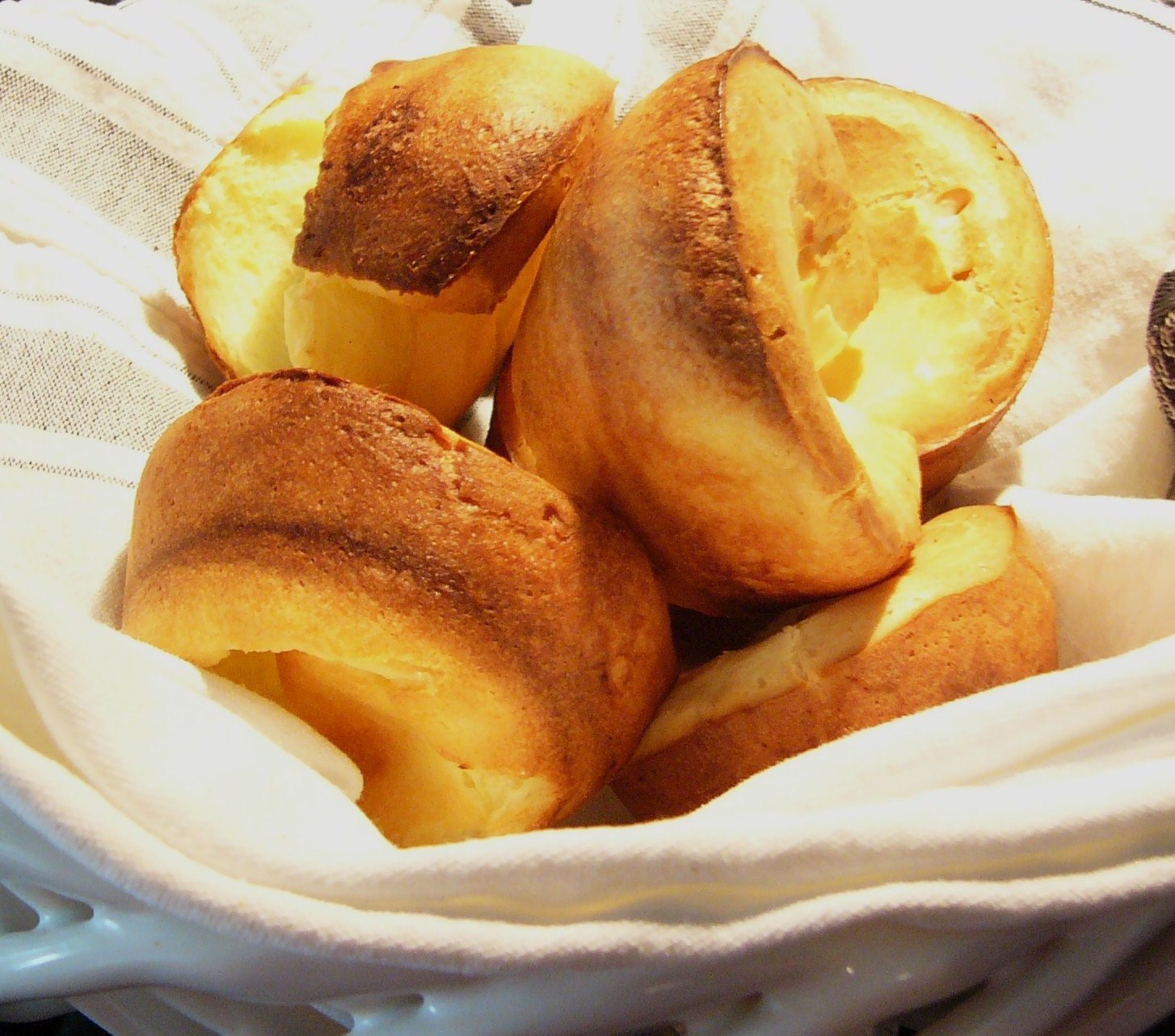A bright, well-lit image captures the warmth and inviting appearance of four small, round pastries nestled in a soft cloth-lined glass basket. These pastries, sporting a golden-brown crust with slightly darker edges, appear untouched and freshly baked. The top-left pastry has an open top, revealing its soft inner texture, while the others resemble torus-shaped buns with nuanced browning, suggesting a crispy, delicate exterior. The basket is lined with a towel accented by a single faded black stripe on the left. Despite their uneven shapes, the pastries collectively create a harmonious display of rustic charm, drawing all attention to their appetizing presentation. The composition focuses solely on the pastries, leaving little room for distraction, capturing their delightful and freshly made essence.